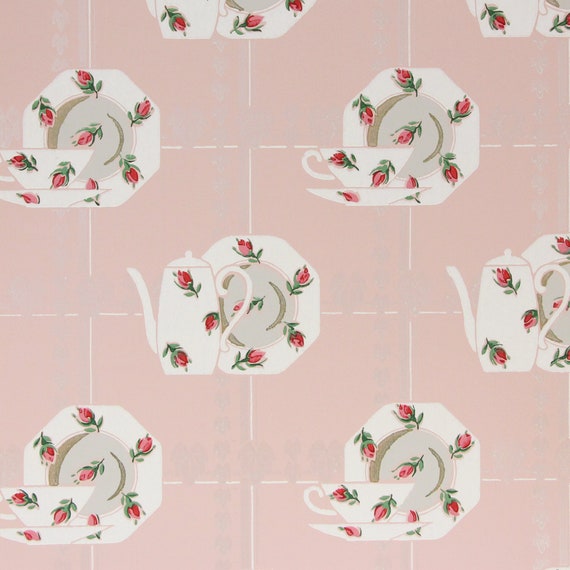The image features a delicate pattern set against a light pink, almost peach-colored background, designed to resemble tiles with dotted lines forming a grid of small squares. At the top left and right, there are white plates adorned with roses along their edges and a single rose in the center. Each plate supports a teacup and saucer, also decorated with a rose pattern. In the middle of the image, there is a teapot featuring the same rose design. Below this, the pattern repeats with another set of plates and teacups. The orderly, alternating arrangement of floral-themed dinnerware captures a sense of symmetry and elegance across the entire image.